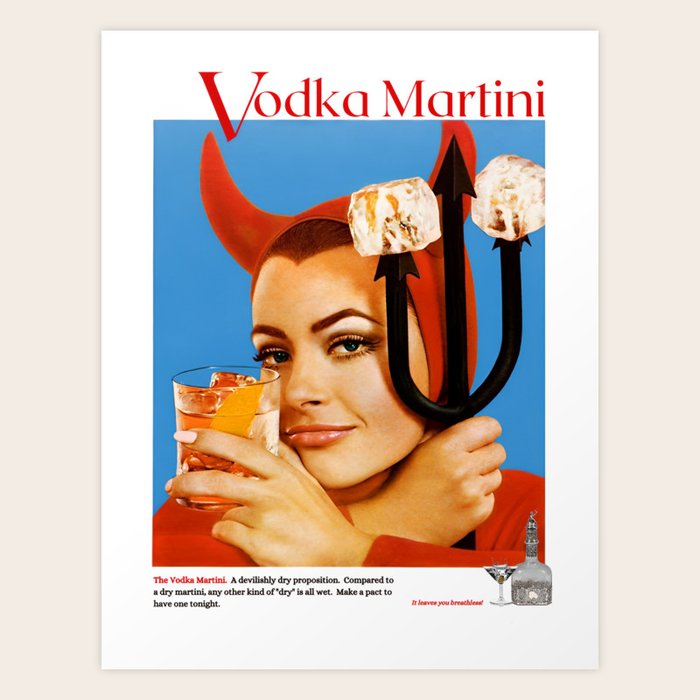This is an old-fashioned advertisement for a Vodka Martini, styled like a product ad from the 1960s or 70s. The ad features a woman dressed in a devil costume, positioned centrally, with only her shoulders and head visible. She wears a red, long-sleeved shirt, a headpiece with red devil horns, and holds a black pitchfork with three prongs. The left side of the image shows her holding a glass of vodka martini garnished with ice and a lemon slice. 

The poster is predominantly white with a gray background. The text at the top reads "Vodka Martini," and at the bottom, it states, "The Vodka Martini: a devilishly dry proposition compared to a dry martini. Any other kind of dry is all wet. Make a pact to have one tonight." The slogan "It leaves you breathless" accompanies an illustration of a vodka bottle and a martini glass. Overall, the ad uses vibrant colors including red, black, and white to create a striking and enticing visual.